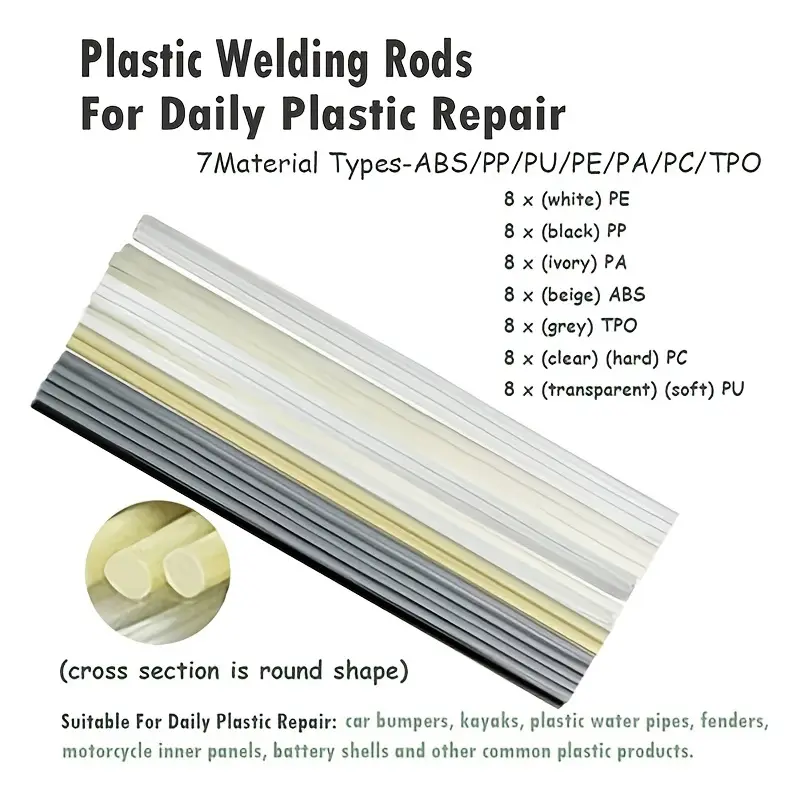**Plastic Welding Rods for Daily Plastic Repair**

The image serves as an infographic for plastic welding rods, titled prominently in dark black font: *"Plastic Welding Rods for Daily Plastic Repair."* It elaborates on the seven material types available: ABS, PP, PU, PE, PA, PC, and TPO. Each type comes in a set of eight units, featuring different colors including white, black, ivory, beige, grey, clear hard, transparent, and soft – each labeled accordingly. A close-up image highlights the round cross-sectional shape of these welding rods, with an annotation stating "cross-section is round shape." The lower part of the infographic details the various applications for these welding rods, such as for repairing car bumpers, kayaks, plastic water pipes, fenders, motorcycle inner panels, battery shells, and other common plastic products. The illustration and text are set against a transparent background, providing a clear and concise visual guide to the product's features and uses.